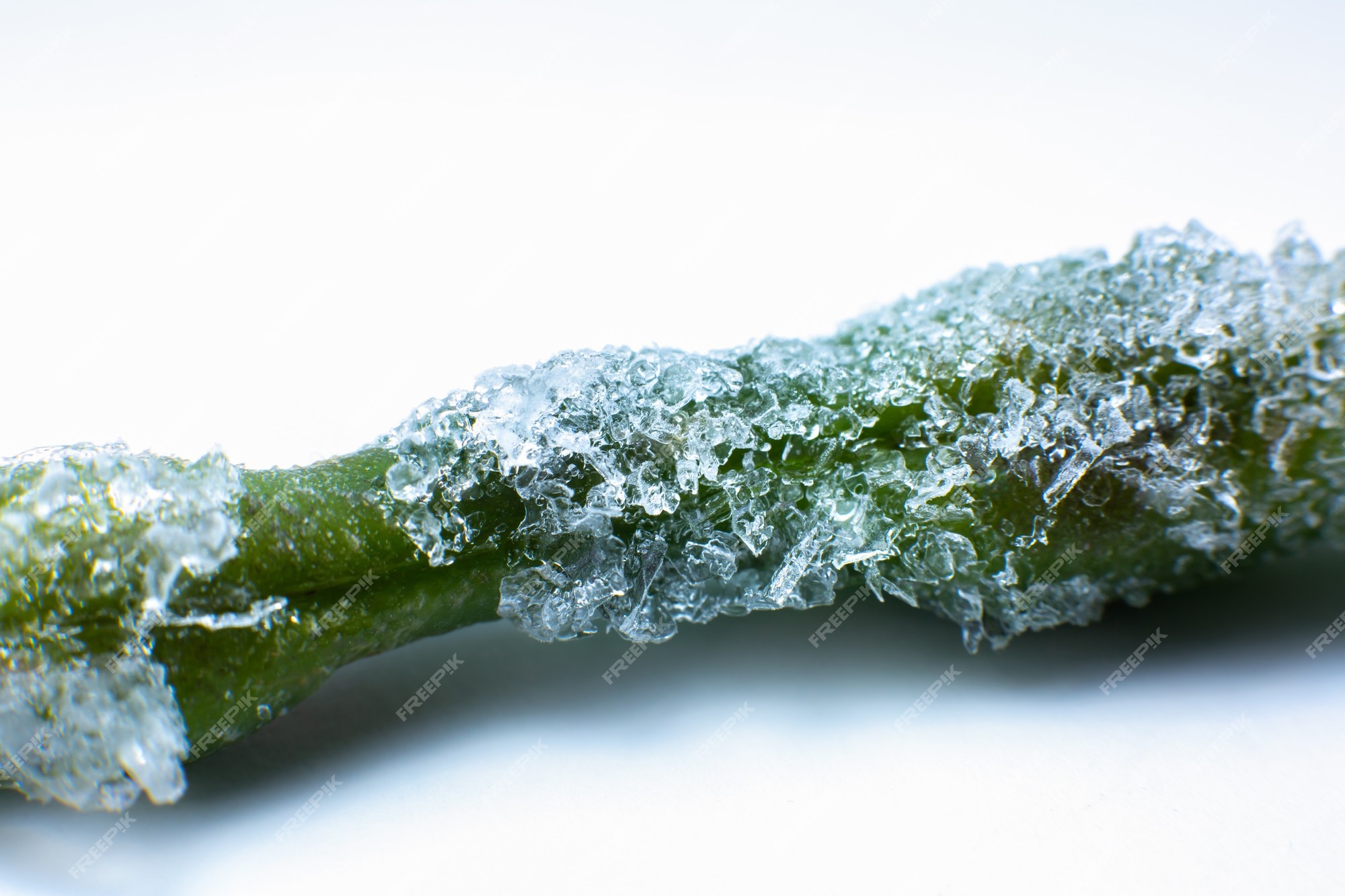The image is a highly zoomed-in photograph of a long, green plant, resembling a cucumber, covered in frozen crystals or frost. This frozen vegetable runs horizontally from the left to the right side of the image, set against a white background with a shadow underneath it. The details are so magnified that the frozen crystals appear almost gelatinous. The entire image is encumbered with watermarks spelling out "Free Pick" (F-R-E-E-P-I-X) in various places, adding a noticeable layer of text over the subject.